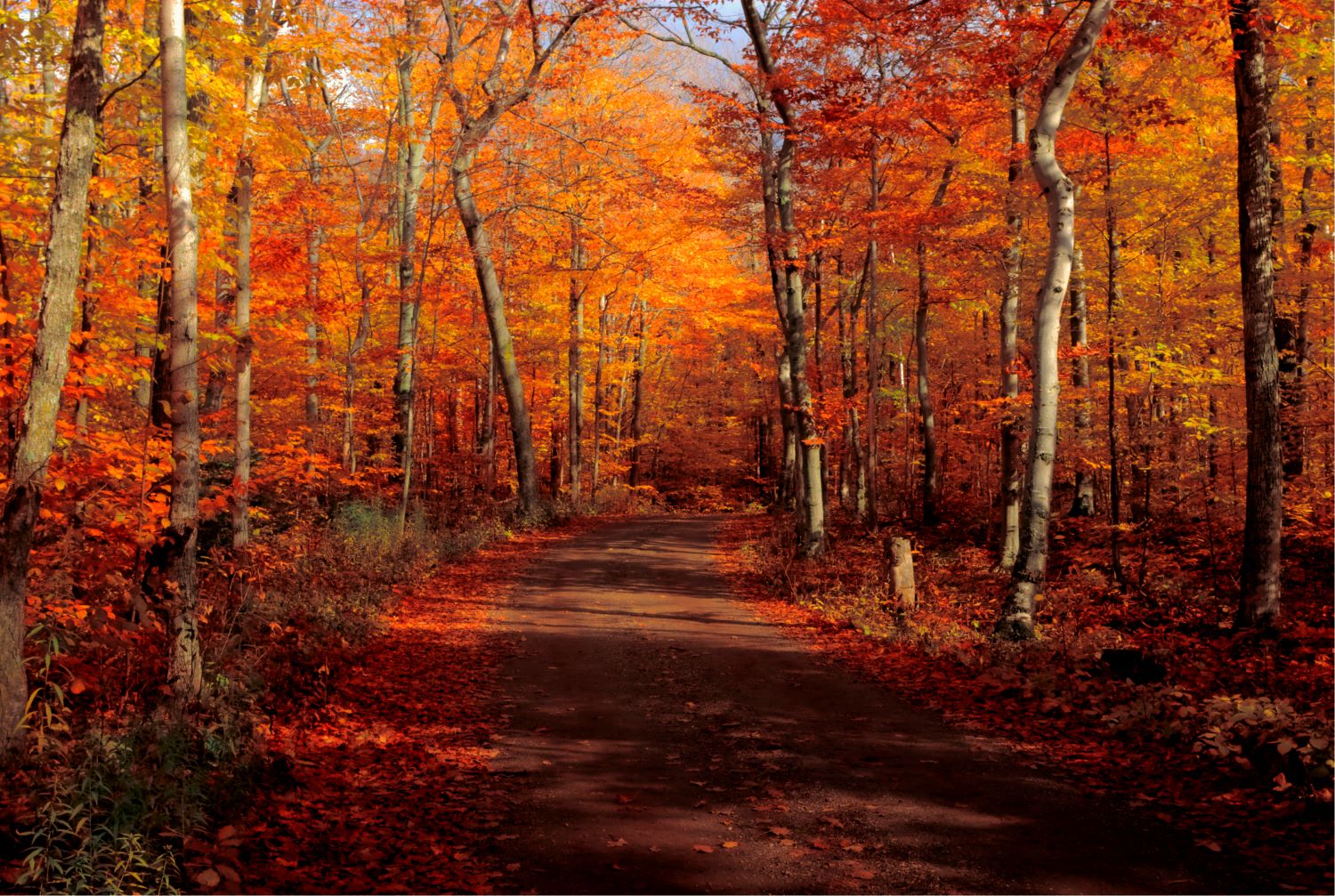This photograph captures a quintessential autumn scene, likely taken in a place reminiscent of Shenandoah National Forest in October. A paved path, gray and soft underfoot, extends down the middle of the frame, inviting a seamless journey through a serene, flat terrain. Tall, thin tree trunks stretch upwards, their branches adorned with vibrant fall foliage in shades of gold, orange, red, and yellow. The ground is carpeted with similarly colored leaves, with only a few scattered on the path itself. Amid the vivid colors, green brush plants and sporadic white pine trees add depth to the landscape. Shadows cast by the trees dapple the path, and a hint of a blue sky peeks through the dense canopy, suggesting a clear, sunny day perfect for a peaceful hike in this forested haven.